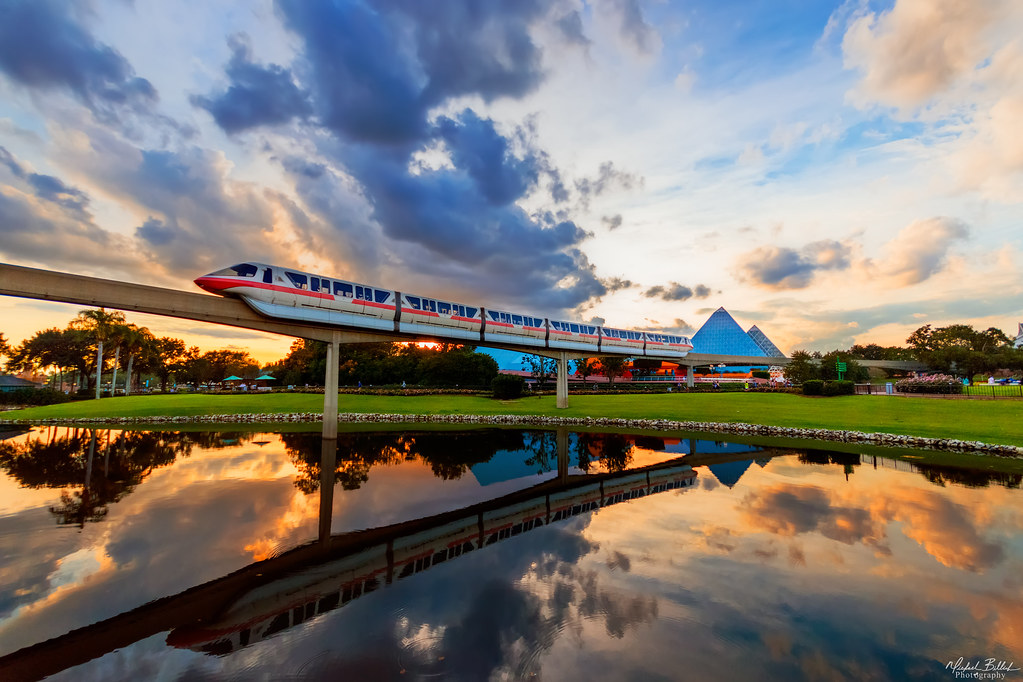This photograph captures a stunning scene, likely in an amusement park setting such as Orlando, Florida, featuring a sleek, futuristic monorail with a silver body and a red stripe, composed of six connected sections. The monorail glides gracefully on an elevated track over a meticulously manicured green field and a reflective lake, creating mirrored images of both the monorail and the vibrant sky above. The sky is a canvas of soft sunset hues—pink, dark blue, and white clouds blending together. In the background, there are distinctive pyramid-like structures, various buildings, trees, and small umbrellas, adding layers of depth to the landscape. The background elements, including bushes and trees, are silhouetted against the bright sunset, contributing to the tranquil ambiance. Notable details include a long line of rocks that separate the lake from the grassy area and a barely visible artist's signature in the lower right corner of the image.